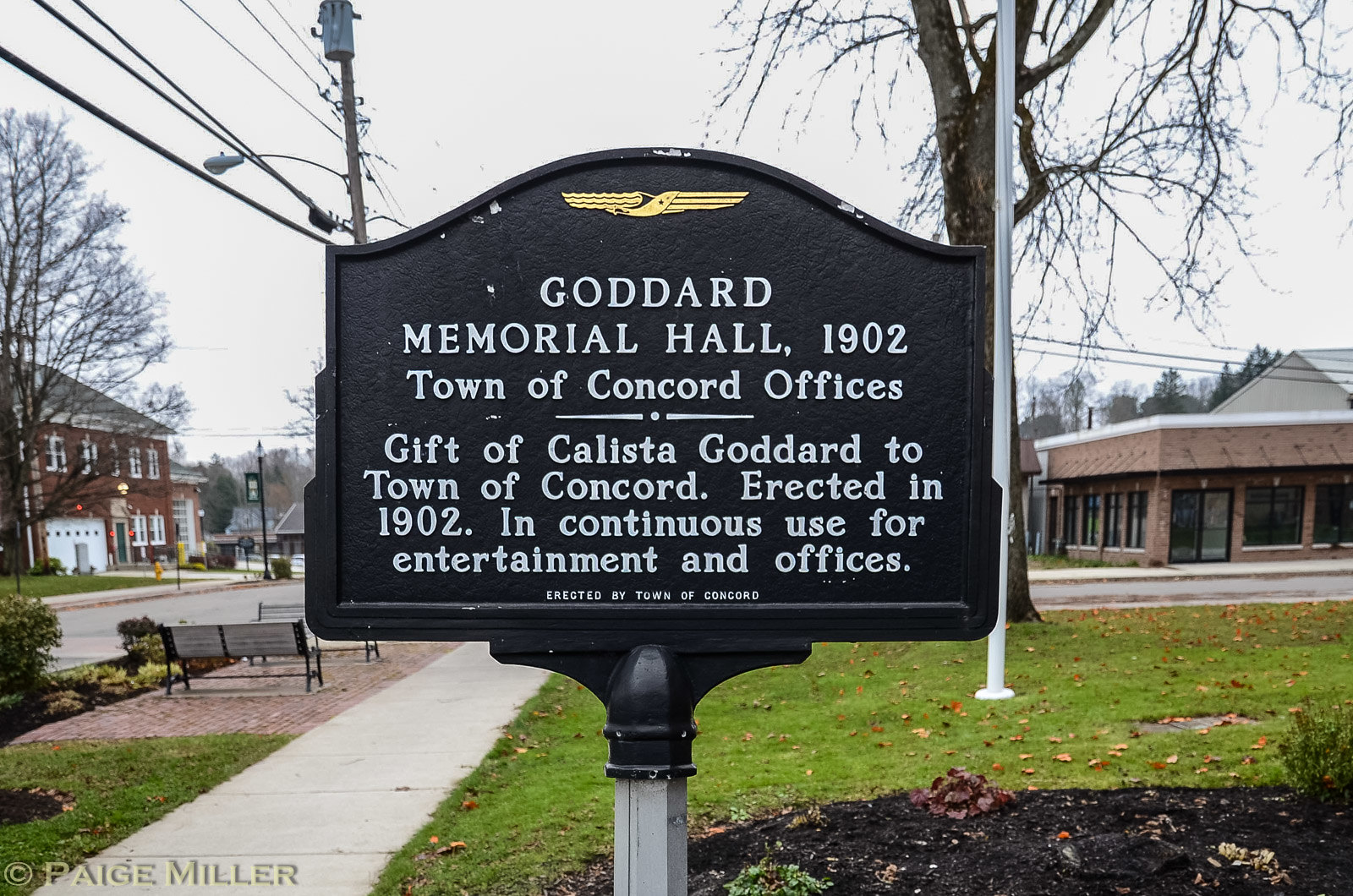The image depicts a black metal sign on an iron post situated on a well-maintained lawn in what appears to be a small town. The sign, with white raised text and an emblem resembling gold wings at the top, reads: "Goddard Memorial Hall, 1902. Town of Concord offices. Gift of Callista Goddard to the Town of Concord, erected in 1902, in continuous use for entertainment and offices. Erected by Town of Concord." The sign shows some white chipping due to age. 

In the left portion of the image, there is a red brick building featuring a white garage door. In this area, a barren tree stands, accompanied by a fire hydrant in front of a sidewalk and lawn. To the left of the plaque, two black benches are positioned near a brick-paved area, offering seating next to the sidewalk. Electrical wires and light posts extend to the upper left of the scene.

A streak of green lawn is visible behind the sign, leading to a white flagpole which stands in front of another barren tree. In the background on the right, another building with lighter brick and windows can be seen, contrasting with the darker brick structure on the left. The overall atmosphere suggests a wet, rainy autumn day, with the trees bereft of leaves but the grass still vividly green.